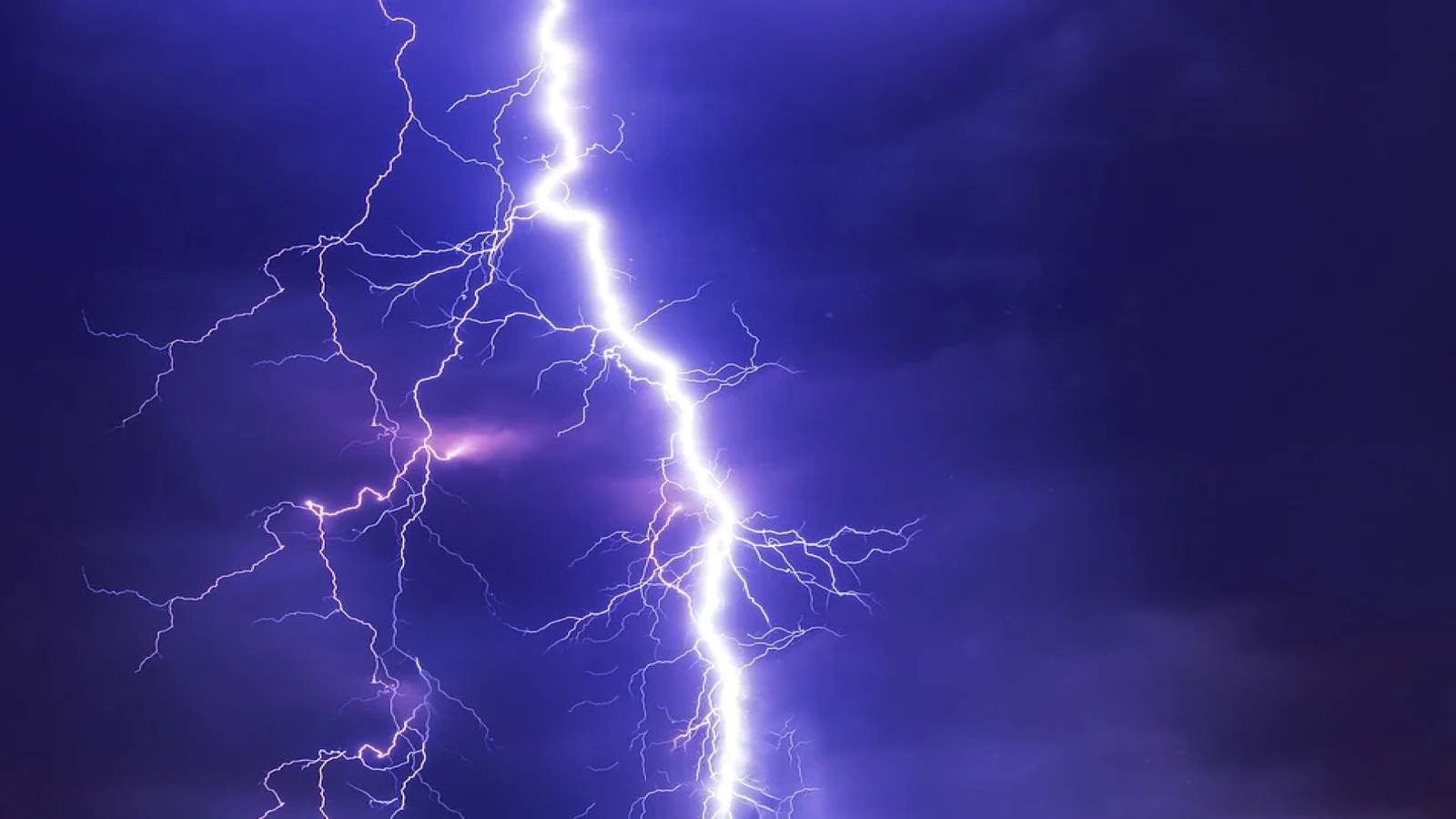This striking photograph captures an intense lightning storm against a dramatic sky. Dominating the image is a thick, bright white, jagged lightning bolt that splits the scene vertically down the middle. This primary bolt, radiant and powerful, is complemented by a thinner but equally energetic lightning strike beside it. The background sky is a mesmerizing blend of fading purple to dark cobalt blue, with vague, whitish-blue clouds adding texture. Subtle branches of additional lightning activity extend outward from the central bolts, crackling with electric energy. The entire composition creates a vivid tableau of raw, natural power, set against a shifting, cloudy sky, possibly veiling faint stars.